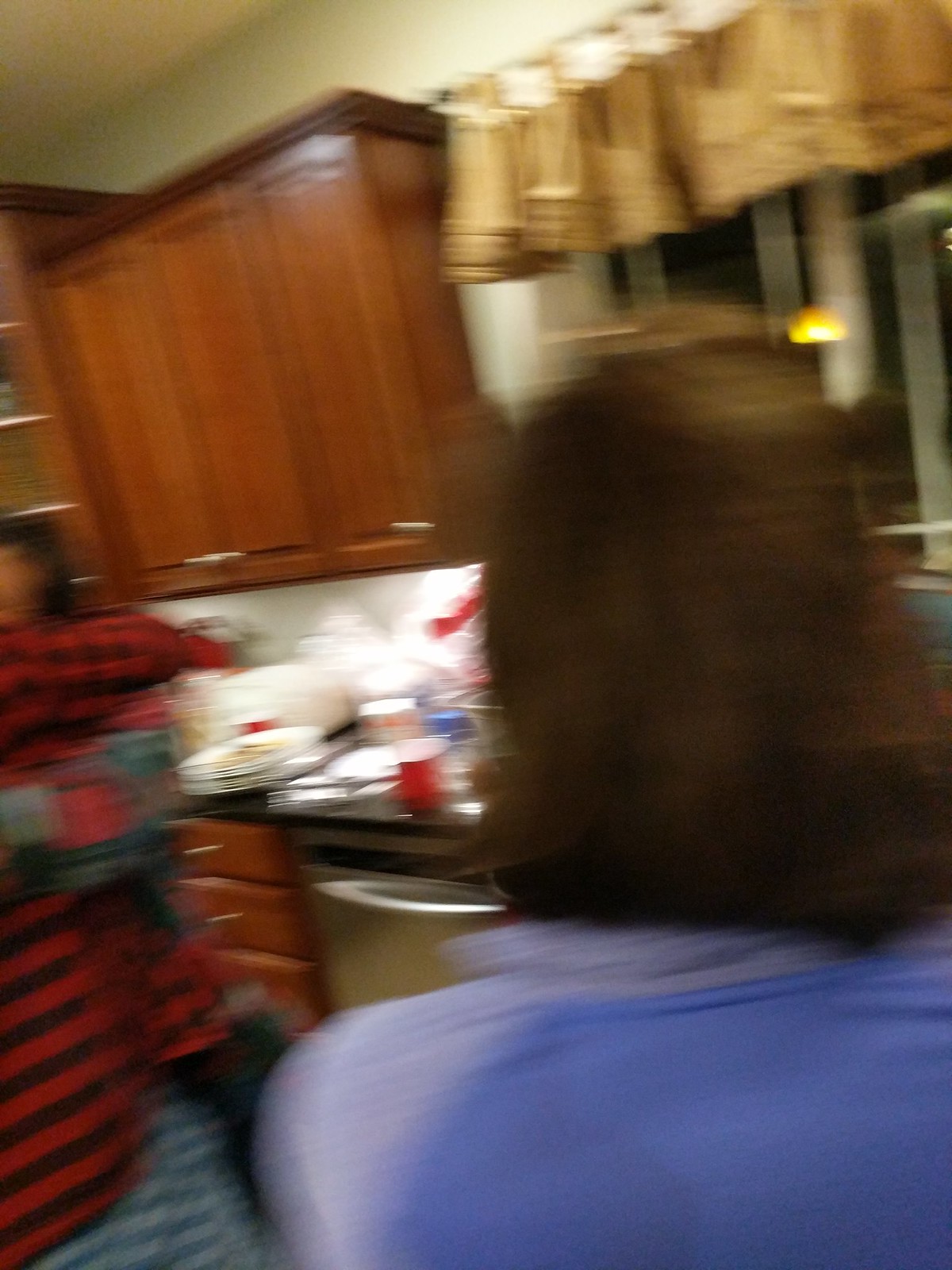The image depicts a cluttered kitchen with a distinct, albeit blurry, scene. At the forefront is the back of a person with shoulder-length hair, likely female, wearing a blue shirt. Off to the left, another individual in a red and black striped shirt is partially visible, with their head cut off in the frame. The kitchen counter is in disarray, covered with various plastic packages, plates, and cups, indicating a messy environment. Below the counter, a dishwasher is discernible along with several drawers. Above the counter, wooden cabinets in a deep brownish hue match the drawer color. To the right of the scene, dark drapes cover a window, suggesting it is nighttime outside. The sink area is not visible, and overall, the image captures a chaotic and untidy kitchen space.